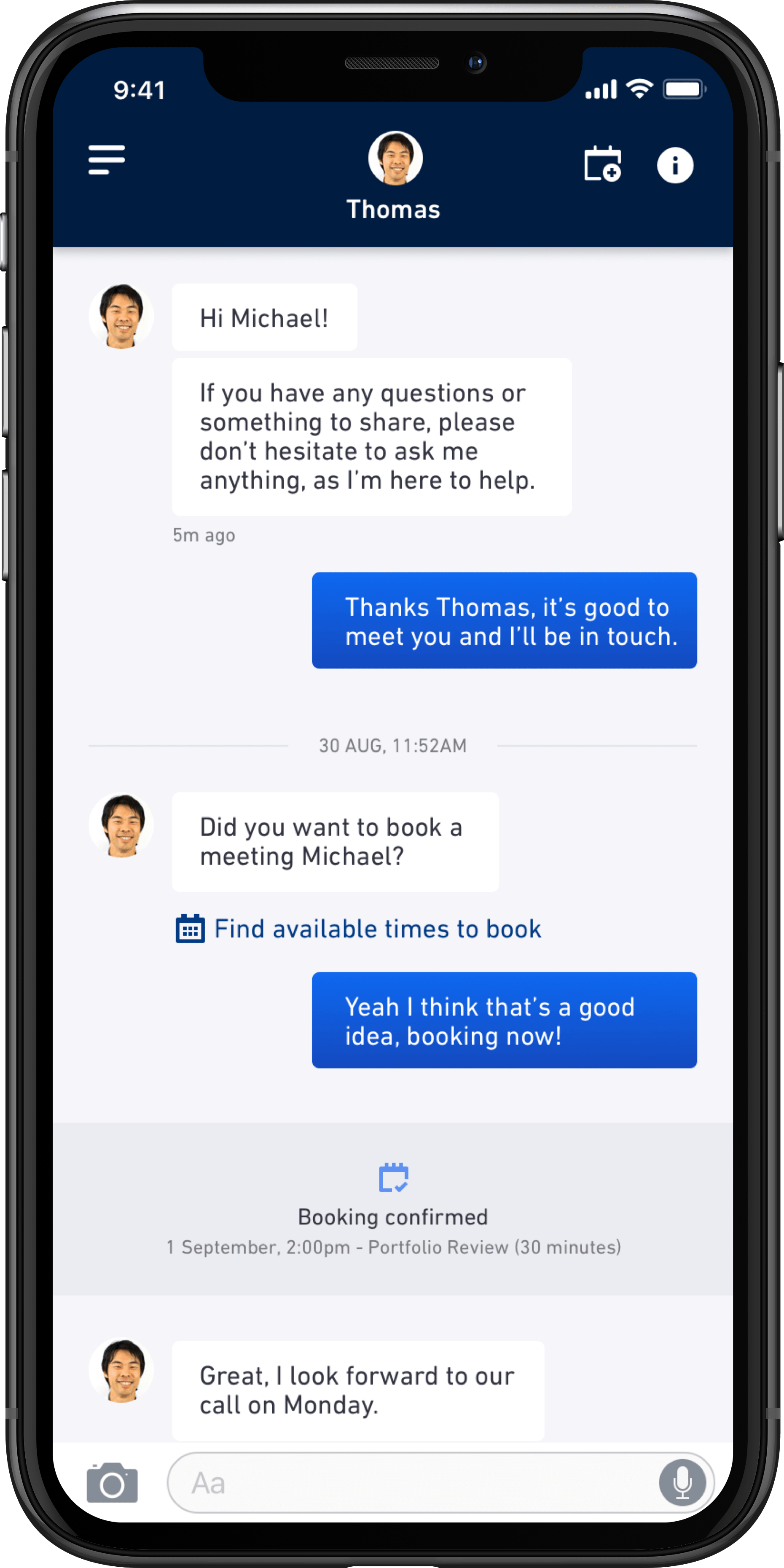This image is a screenshot of a cell phone's messaging application interface. The time displayed at the top of the screen is 9:41, accompanied by full battery and connectivity icons to indicate a strong signal with three bars. On the left side of the screen, a circular profile picture of a man is visible, identified as "Thomas" by the text below the image in white print. To the right of his name, there is an additional application icon and a lowercase "i" enclosed in a white circle, possibly for information or settings access.

The conversation visible in the screenshot shows an exchange between Thomas and another person named Michael. Thomas starts the conversation by saying, "Hi Michael, if you have any questions or something to share, please don't hesitate to ask me anything as I'm here to help." In response, Michael writes, "Thanks Thomas, it's good to meet you and I'll be in touch." 

A gray line draws attention to a timestamp indicating "30 August, 11:52 a.m." Thomas then follows up with, "Did you want to book a meeting, Michael?" and suggests looking for available times to book the meeting. The conversation concludes with Michael agreeing, saying, "Yeah, I think that's a good idea. Booking now."